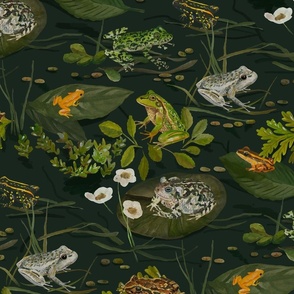The image is an illustration of a vibrant pond teeming with life. The scene features a multitude of green lily pads and various leaves that float serenely on the water's surface. The leaves come in different shapes and sizes, with some being large and round while others are teardrop-shaped. Scattered across these leafy platforms are numerous frogs of varying sizes and striking colors. These frogs exhibit a remarkable array of patterns and hues, including solid white, bright orange, black and orange stripes, green with brown stripes, and more complex combinations like white with black dots and green with black dots. There's even a frog with white and black markings. The detailed depiction suggests the use of oil paint or markers. Notably, one frog on a dark green leaf in the bottom right corner is particularly vivid in orange with a distinctive black eye, while a nearby frog displays a brown-yellow coloration with black eyes. The overall artwork is a cohesive, square-shaped composition, likely hand-drawn or painted, illustrating a richly populated and diverse aquatic ecosystem.